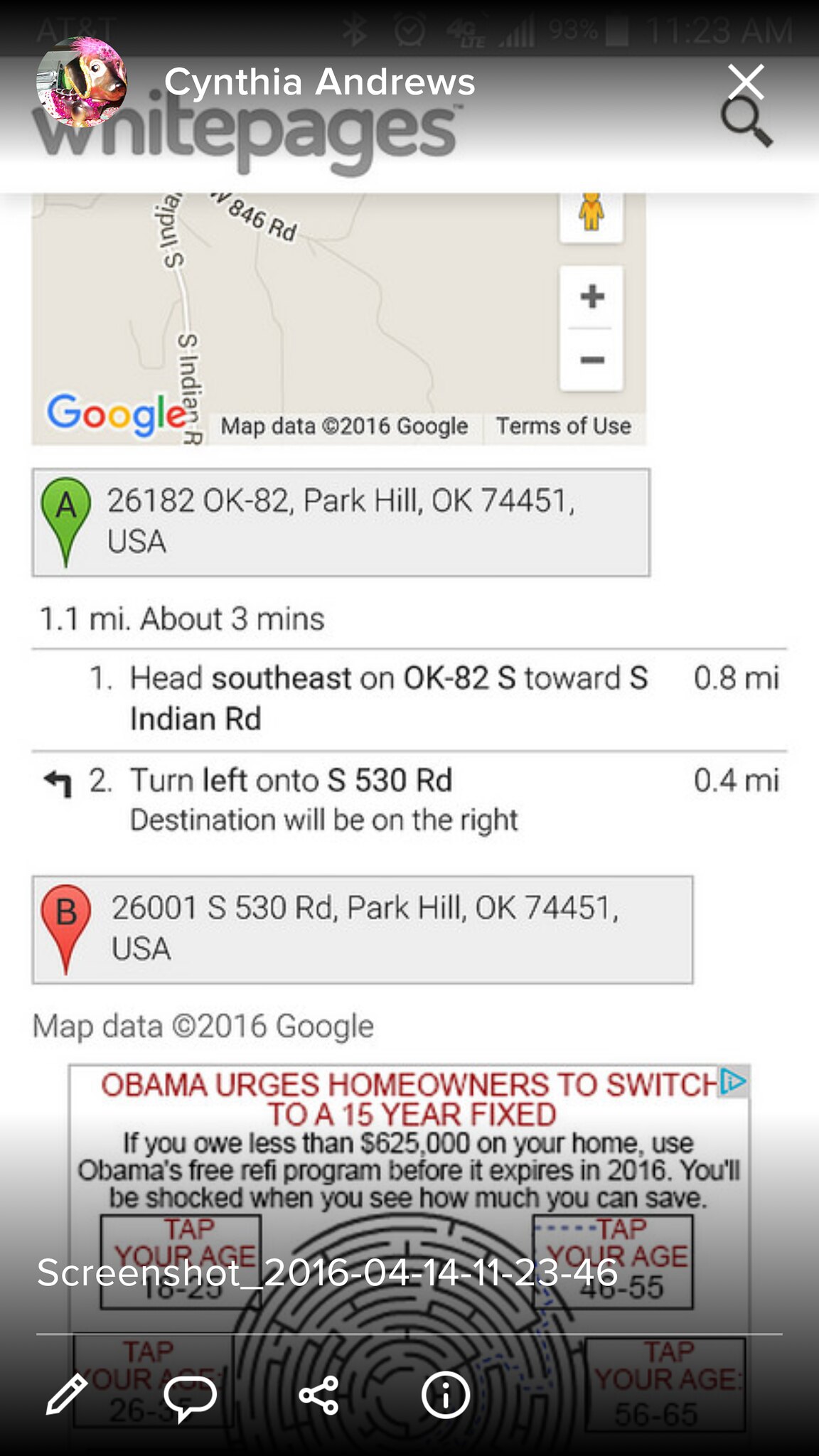This image is a screenshot from either Whitepages.com or the Whitepages mobile app, as indicated at the bottom of the image. At the top of the screenshot, there is a profile for someone named Cynthia Andrews, complete with an avatar, which resembles the layout of an Instagram account. This might suggest that the screenshot was taken from a social media post or shared on an Instagram account by Cynthia.

The main portion of the image is dominated by a Google Map. It shows directions starting from an unspecified address on Highway 82 in Park Hill, Oklahoma. The route detailed by Google Maps includes a southeast turn and a left turn, leading to an unspecified location on South 530 Road in Park Hill. The directions suggest that it only takes about three minutes to reach the destination, which might imply a short, local trip, potentially to a private address that is not explicitly detailed in the image.

At the bottom of the screenshot, beneath the Google copyright information, there's an advertisement. This ad is about former President Obama urging homeowners to switch to a 15-year fixed mortgage rate, complete with a chart illustrating the potential risk associated with different mortgage terms. The ad and its content suggest that the screenshot was most likely taken in 2016.

Overall, this screenshot captures navigation directions coupled with an ad, suggesting it might have been shared on social media for a specific informative purpose.